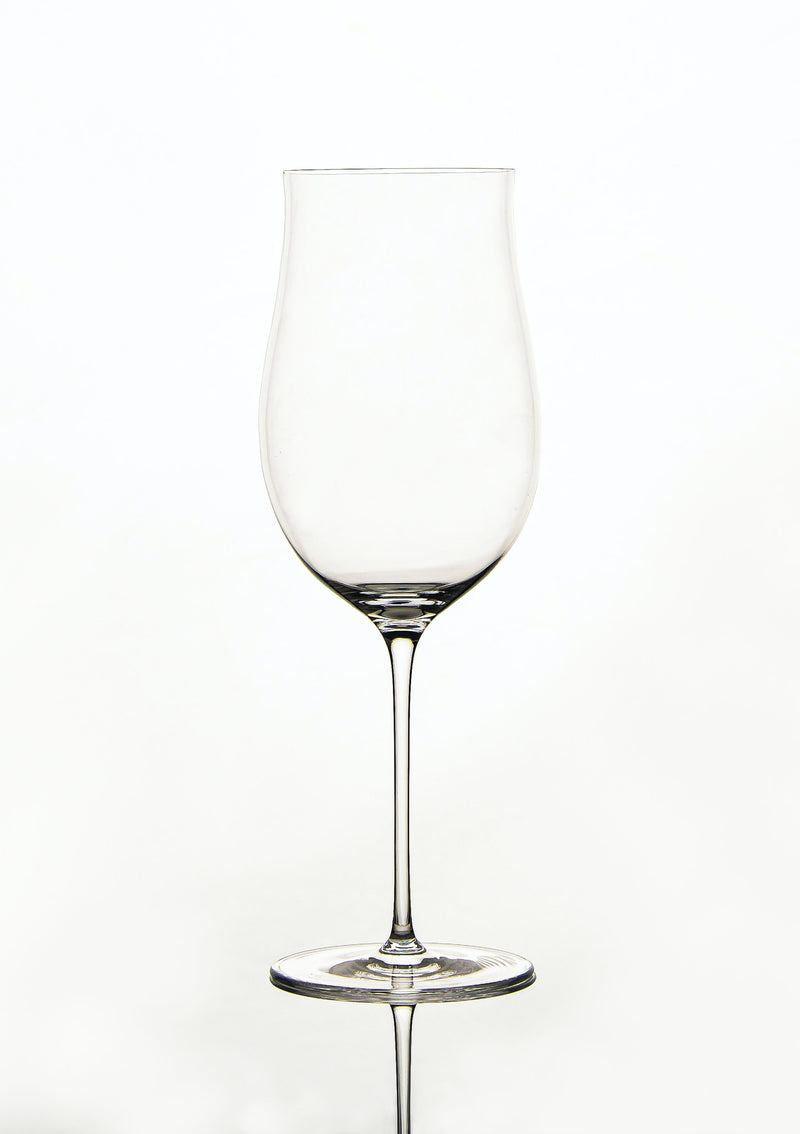The image features a clear wine glass with a thin, narrow stem that is approximately four to five inches tall. The bowl of the glass flares out slightly at the bottom and then tapers toward the top, giving it a fluted shape. The wine glass is empty, without any liquid inside. The glass is either standing on a reflective surface or an identical upside-down glass, creating the illusion of a reflection or a stacked arrangement. The background of the image is solid white, and the image itself is vertically oriented and rectangular in shape. There's no text or additional colors in the image, focusing solely on the clear glass.